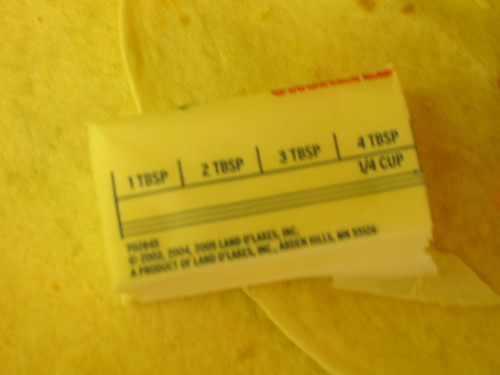In the image, a partially unwrapped stick of butter, marked with tablespoon measurements, rests atop two neatly stacked flour tortillas. The butter, encased in its recognizable paper wrapper, appears slightly used, suggesting it’s ready to enhance the flavor of the soft, warm tortillas underneath. This nostalgic setup evokes memories of childhood, where a simple yet delightful snack of warm tortillas spread with melting butter was a cherished treat.